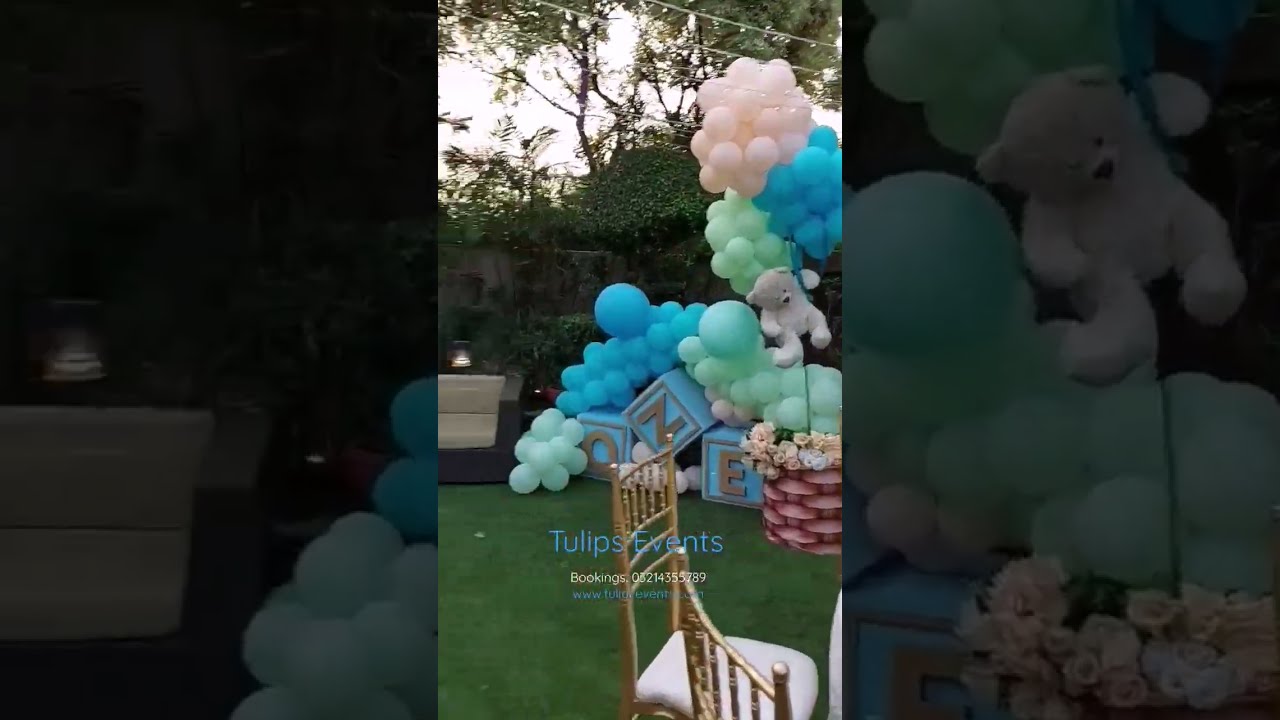The image depicts a vibrant birthday celebration set in a well-maintained backyard. The scene features lush green grass, several trees, and a stone wall in the background. There are string lights overhead adding a festive ambiance. Central to the display are three large blue blocks with gold trim, each bearing a gold-lettered "O," "N," or "E." These blocks are artistically arranged with the "O" flat on the ground, the "N" leaning at an angle, and the "E" upright. Surrounding the blocks are bunches of colorful balloons in green, blue, pink, and white, with a white teddy bear seemingly clinging to one of them.

Additionally, there is a sophisticated outdoor setup including an ornate gold and cream fabric chair, a matching table and chairs ensemble, and an outdoor sofa. Decorative elements like a basket with white and pink flowers enhance the celebratory atmosphere. The image features a blue text overlay that reads "Tulips Events Bookings," with a contact number (032-143-55789) and the website www.tulipsevents.com, indicating it is an advertisement for an event planning company.